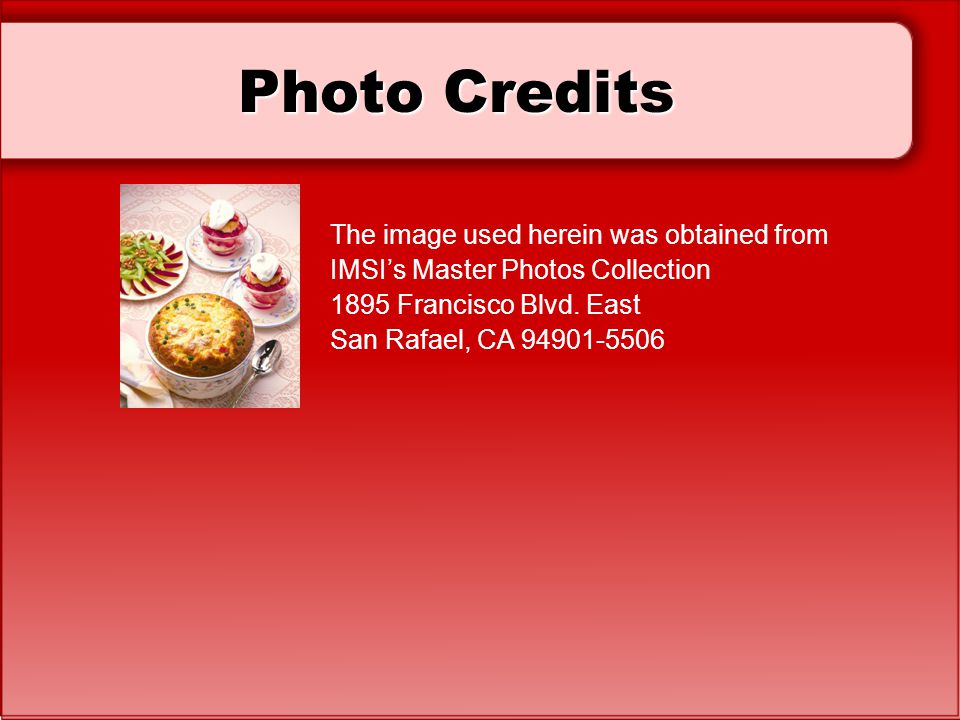The image depicts a slide from a presentation, specifically a photo credits slide, featuring a red background with a gradient transitioning from a darker red at the top to a lighter red at the bottom. At the top, a pink rectangular panel spans almost the entire width of the slide, containing the title "Photo Credits" in black font, with a very slight white border around the letters. Beneath this, there is a centrally positioned image showcasing an assortment of desserts: two parfaits topped with whipped cream in clear glass dishes on a saucer, a decorative arrangement of apple slices with green garnish, and what appears to be a baked dessert, possibly a quiche or souffle, in a ceramic ramekin accompanied by a silver spoon. To the right of the dessert image, white text provides the photo source information: "This image used herein was obtained from IMSI's Master Photos Collection, 1895 Francisco Boulevard East, San Rafael, California, 94901-5506."